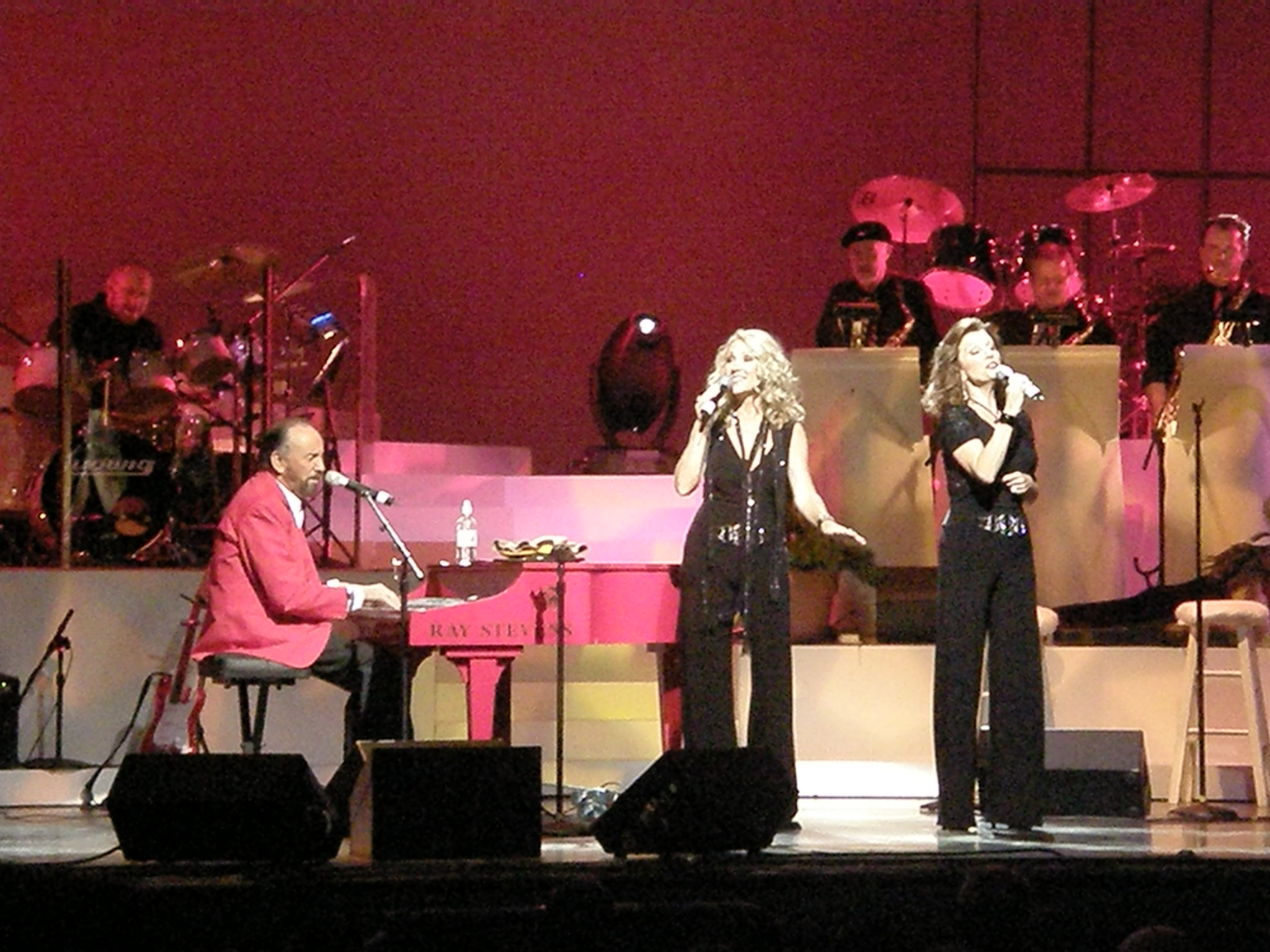The image captures a vibrant performance on a raised stage with a black surface, featuring multiple musicians. Front and center, two women are passionately singing into microphones, both clad in black pants and coordinating black belts. The woman on the right wears a short-sleeved V-neck top and a black necklace, while the woman on the left sports a sleeveless tank with a low V-neck. The singers, identified as a brunette and a blonde, exude energy and harmony.

To their left, a man in black pants and a distinctive pink coat with a white button-up shirt is seated at a pink piano on a foldable black bench. A water bottle rests on top of the piano. This man is part of Ray Stevens' band, as indicated by text nearby.

Behind the singers, the elevated platform houses the drummer, who is encased in glass and dressed entirely in black. Also on the stage are several other band members playing wind instruments, including what appears to be trombones, adding layers to the musical performance. The stage setup includes multiple speakers aimed at the performers, ensuring their sound reaches the audience clearly.